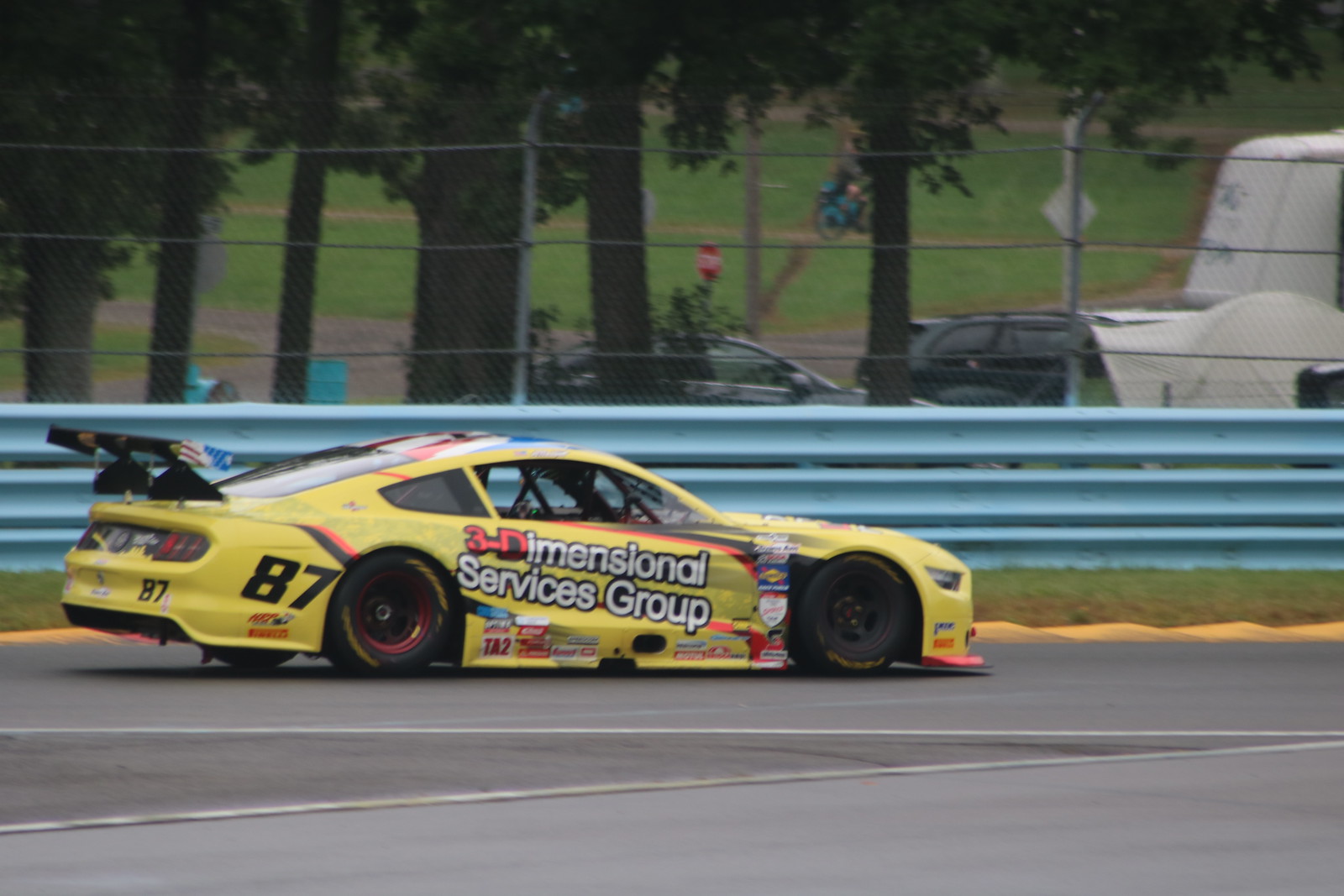The image showcases a vibrant yellow race car, prominently featuring the black number 87 positioned just behind its back passenger wheel. The car sports a sponsor logo in white text that reads "Three Dimensional Services Group," accompanied by a red "3D" on the door, accentuated by black and red stripes nearby. The race car is on a cement raceway bordered by a light blue guardrail, with a grassy verge and a yellow cement border further illustrating the track's edge. In the background, one can observe a higher blue fence, likely a chain-link type, which separates the raceway from a road or additional service path. Visible beyond the blue fencing is a grassy area with trees, a cyclist or motorcyclist, and several parked vehicles, including a black SUV and a white van. This detailed backdrop provides a lively context to the vibrant scene captured on the racetrack.